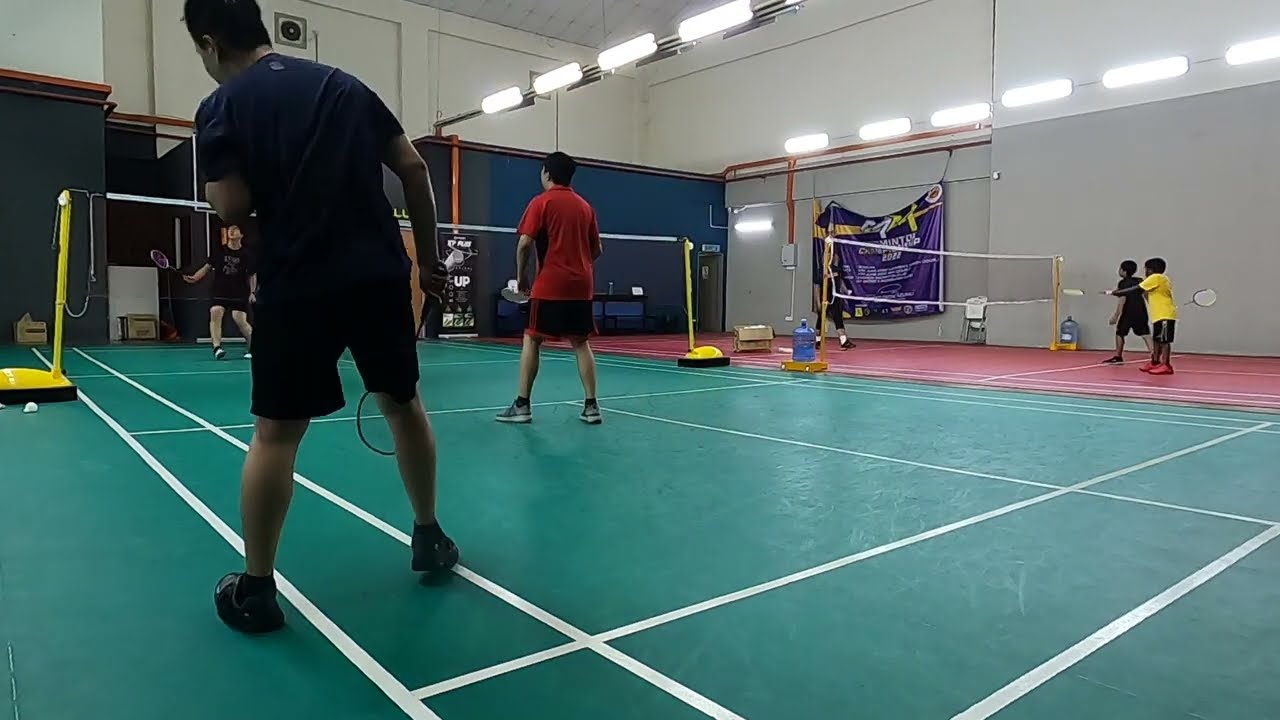The image captures an indoor scene of a vibrant badminton game featuring two small adjacent courts within a tall-ceilinged building. Closest to the camera is a green court, outlined with white stripes, where three young men are intensely engaged in playing badminton. The player nearest to us, with dark short hair, is dressed in a blue top and black shorts, holding a racket. Slightly further away stands another player in a red t-shirt and black and red shorts, while the third player across the net, in black attire, looks upward, likely tracking the shuttlecock's flight. The green court is divided by a white net supported by yellow stands with black bases, and a shuttlecock is visible near one of the stands.

Adjacent to the green court is a red court, also lined with white stripes, where three younger players—two girls—are playing. One girl is in a bright yellow t-shirt, and the other is primarily in black. Both courts reside within a building that features white walls and gray upper sections, decorated with a large purple banner advertising a "Badminton Championship 2022" in white and yellow text. The lighting is provided by rectangular fixtures hanging from the high ceiling, casting a uniform brightness over the courts. In the distant background, a greenish-blue wall gives way to more gray walls, adding to the overall lively yet organized atmosphere of the badminton venue. Stacked jugs of water can be seen holding up the net on the right-hand side of the image.